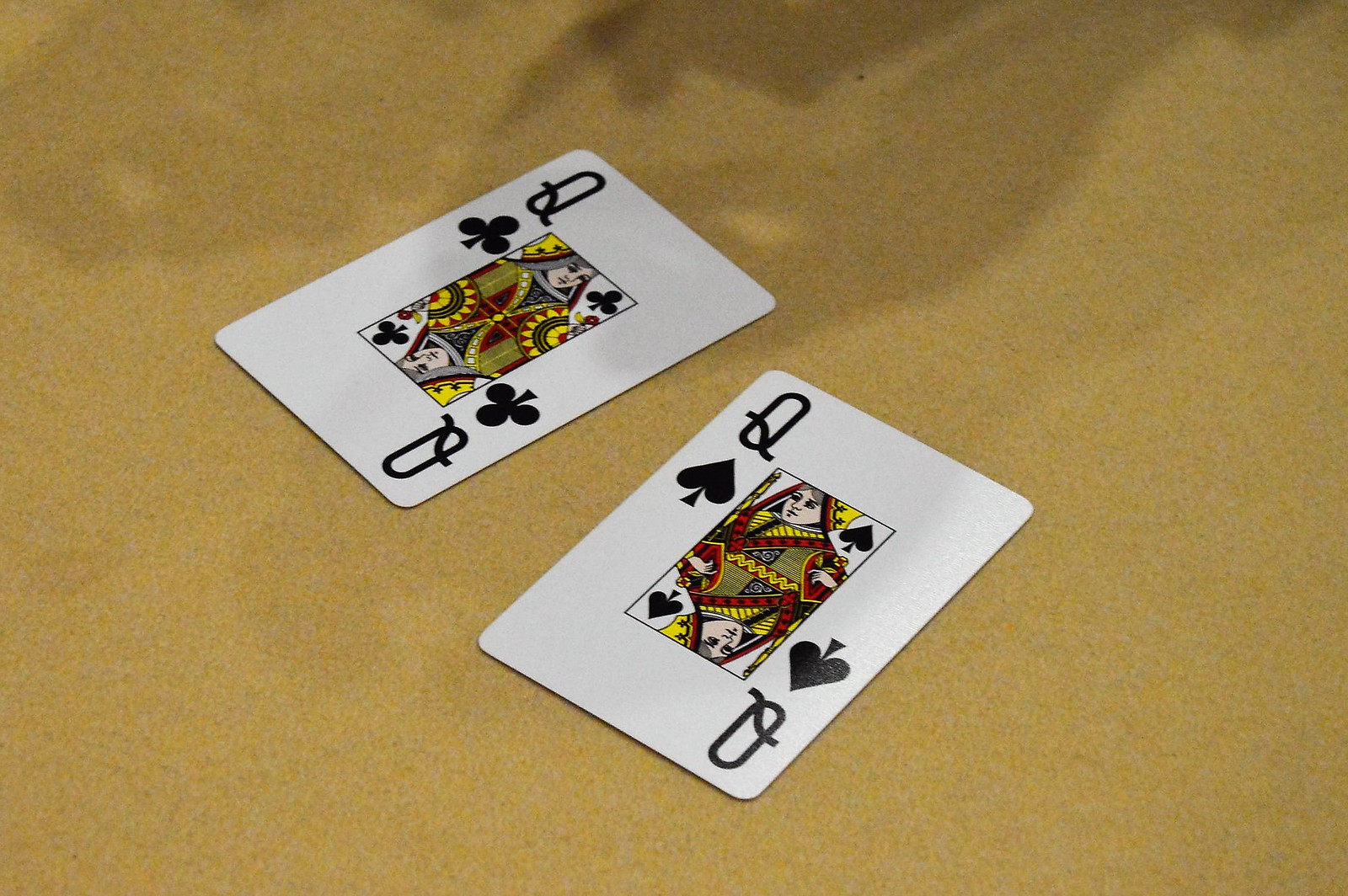In the center of the image, two playing cards are prominently displayed on a tan table. The cards, slightly tilted from the upper right to the lower left, do not touch one another. On the left is the Queen of Clubs, marked by a large "Q" in the corners, with the club symbols positioned at the top left and bottom right. On the right is the Queen of Spades, featuring a similarly large "Q" in the corners, with the spade symbols in the same arrangements.

Both Queens are depicted in medieval attire within a small rectangle in the center of each card, adorned in a rich palette of reds, yellows, light greens, blacks, and whites. The intricate detailing of their garb adds to the card's classic allure. A shadow crosses the upper right side of the image, cutting through the Queen of Clubs and extending towards the top right section of the photograph, adding depth to the scene.